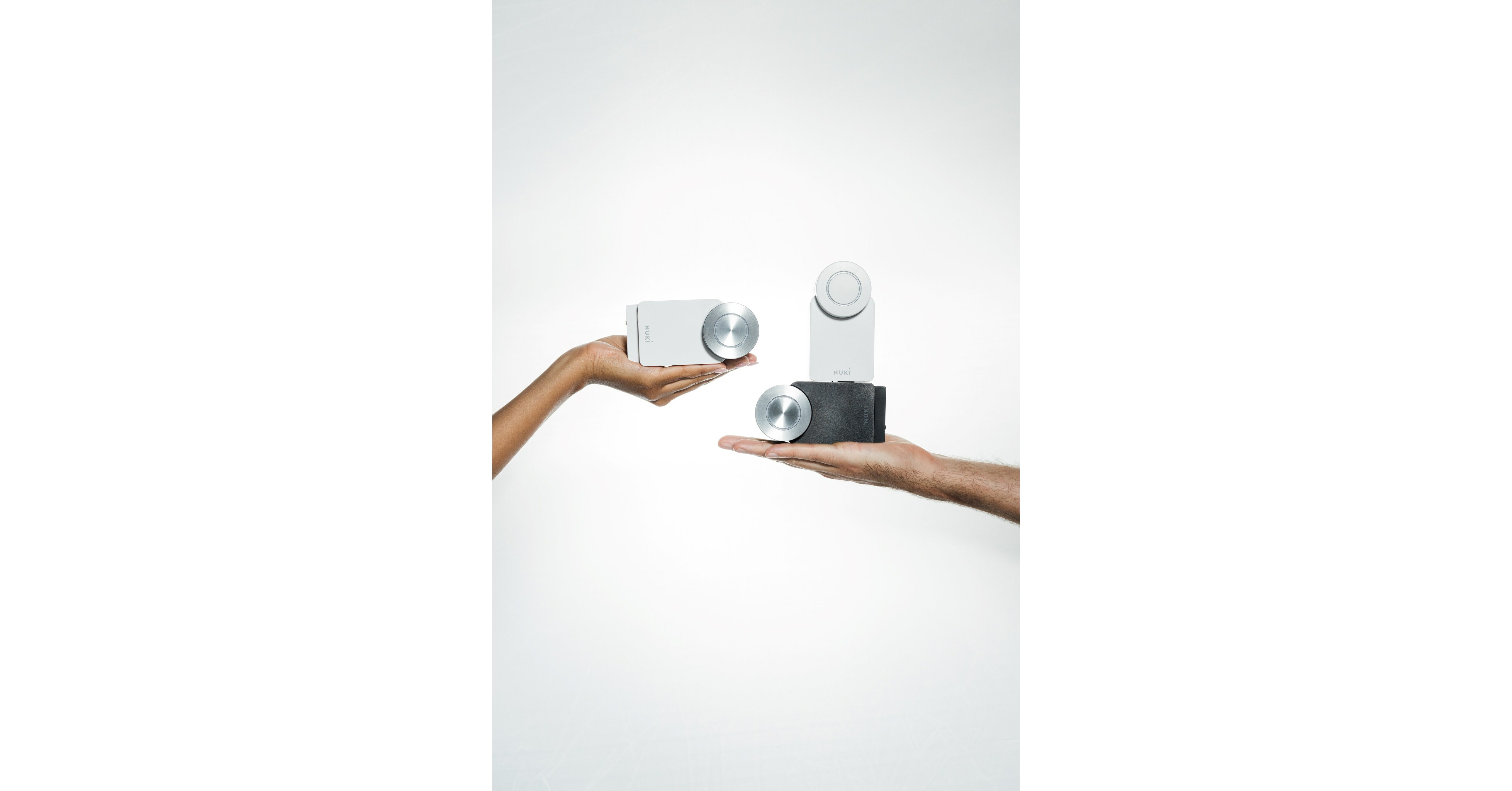The image features a stark white background against which two Caucasian hands—one male and one female—are prominently displayed. Each hand is holding an unusual, indistinct device that resembles the shape of a DSLR camera but is equipped with circular metal rings near one end. The male hand on the right is holding two identical devices, one black and one white, while the female hand on the left holds just one white device. Both devices have a metallic circular component, suggesting they could be used for some unknown function. The lack of context and description leaves the purpose of the devices a mystery, contributing to the bland and uninformative nature of the photo, akin to an uninspiring product listing that fails to engage potential buyers.